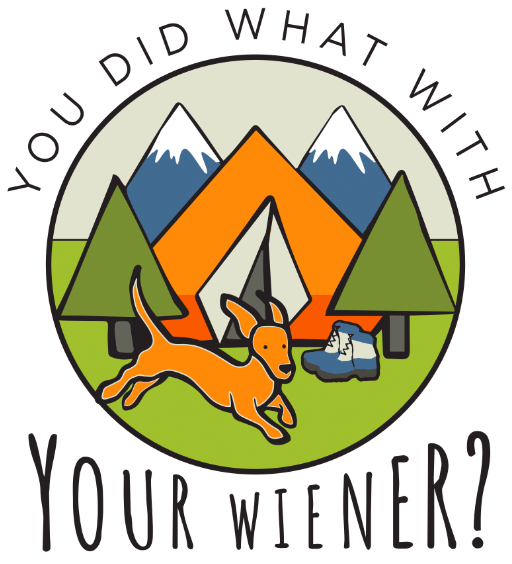This image is a playful, modern, illustrative logo featuring a circular design. At the top of the circle, in black Helvetica all-caps text, it reads "YOU DID WHAT WITH," while the bottom of the circle, in a handwritten all-caps font, continues with "YOUR WIENER?" Inside the circle, a cartoon-style scene unfolds: a brown wiener dog with its ears flying back runs energetically in front of an orange tent with gray flaps. To the right, behind the dog, stands a pair of blue and white hiking boots, and on either side of the tent are two green pine trees with brown trunks. In the background, two triangular blue mountains with snowy white tips complete the fun and whimsical outdoor setting.